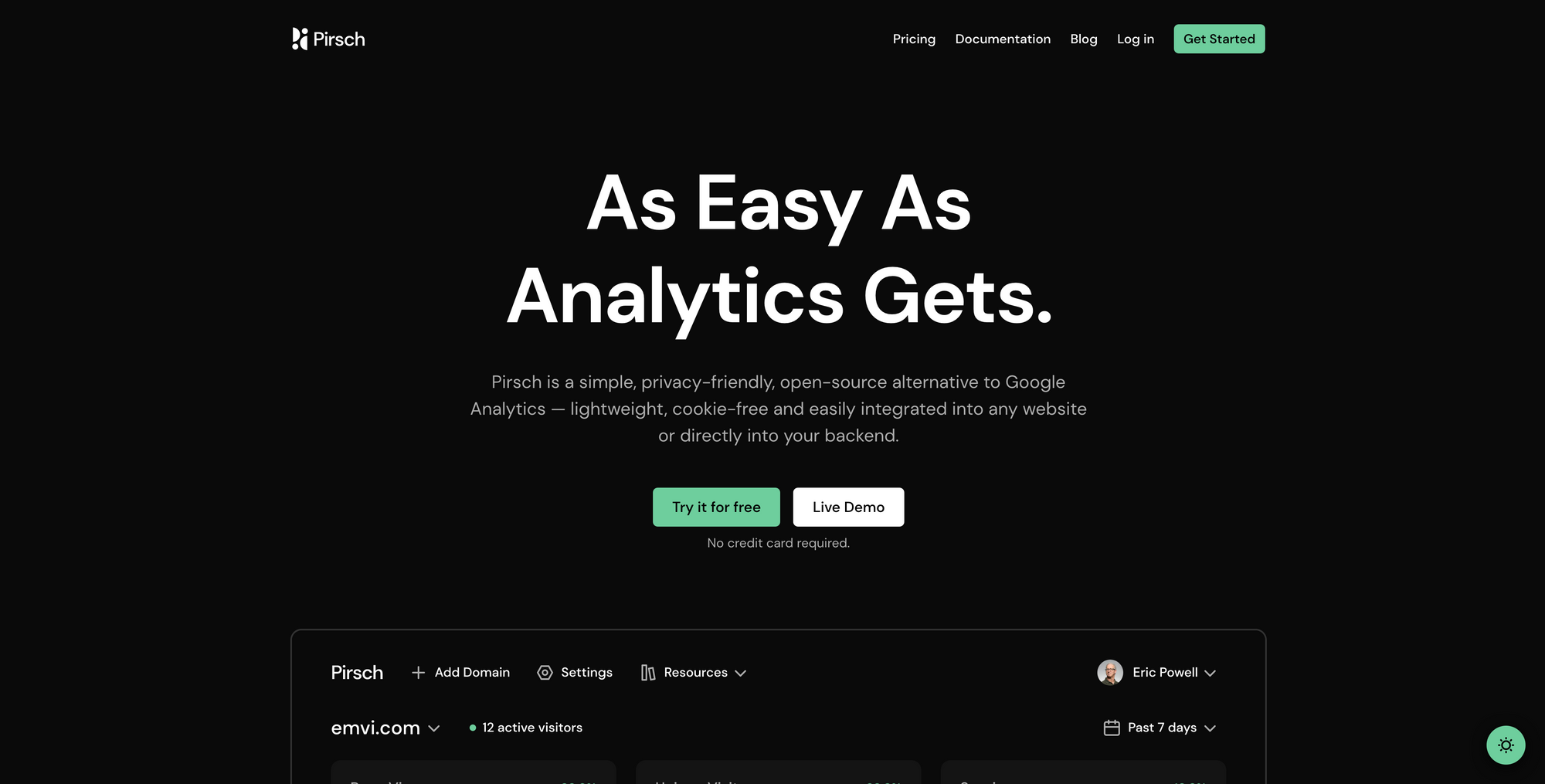This image showcases a webpage for an analytics company named PIRSH. The top section features a black, rectangular banner adorned with a company emblem consisting of half circles and dots, alongside the name "PIRSH" in white letters. To the right of the banner, navigational categories are listed: Pricing, Documentation, Blog, Login, and a prominent green rectangle labeled "Get Started."

The main body of the page has a black background with predominantly white text and certain sections highlighted in black squares with contrasting white lettering. Prominently displayed in the upper center are the words, "As easy as analytics get, PIRSH is a simple, privacy-friendly, open-source alternative to Google Analytics. Lightweight, cookie-free, and easily integrated into any website or directly into your backend."

Below this central message, two action buttons are visible: a green rounded rectangle that reads "Try for Free" and a white rounded rectangle labeled "Live Demo." An additional note reads, "No Credit Card Required."

Lower down, the top portion of another screen is visible, displaying several interface elements including the PIRSH logo, and options for Add Domain, Settings, and Resources. A user account marked "Eric Powell" includes a small circular image placeholder and a timeframe dropdown set to the past 7 days. On the left side, a section labeled "emvi.com" with a dropdown menu shows there are 12 active visitors. A green circular icon appears at the bottom right of the image. The overall design elements emphasize simplicity, ease of use, and privacy-friendly analytics solutions.